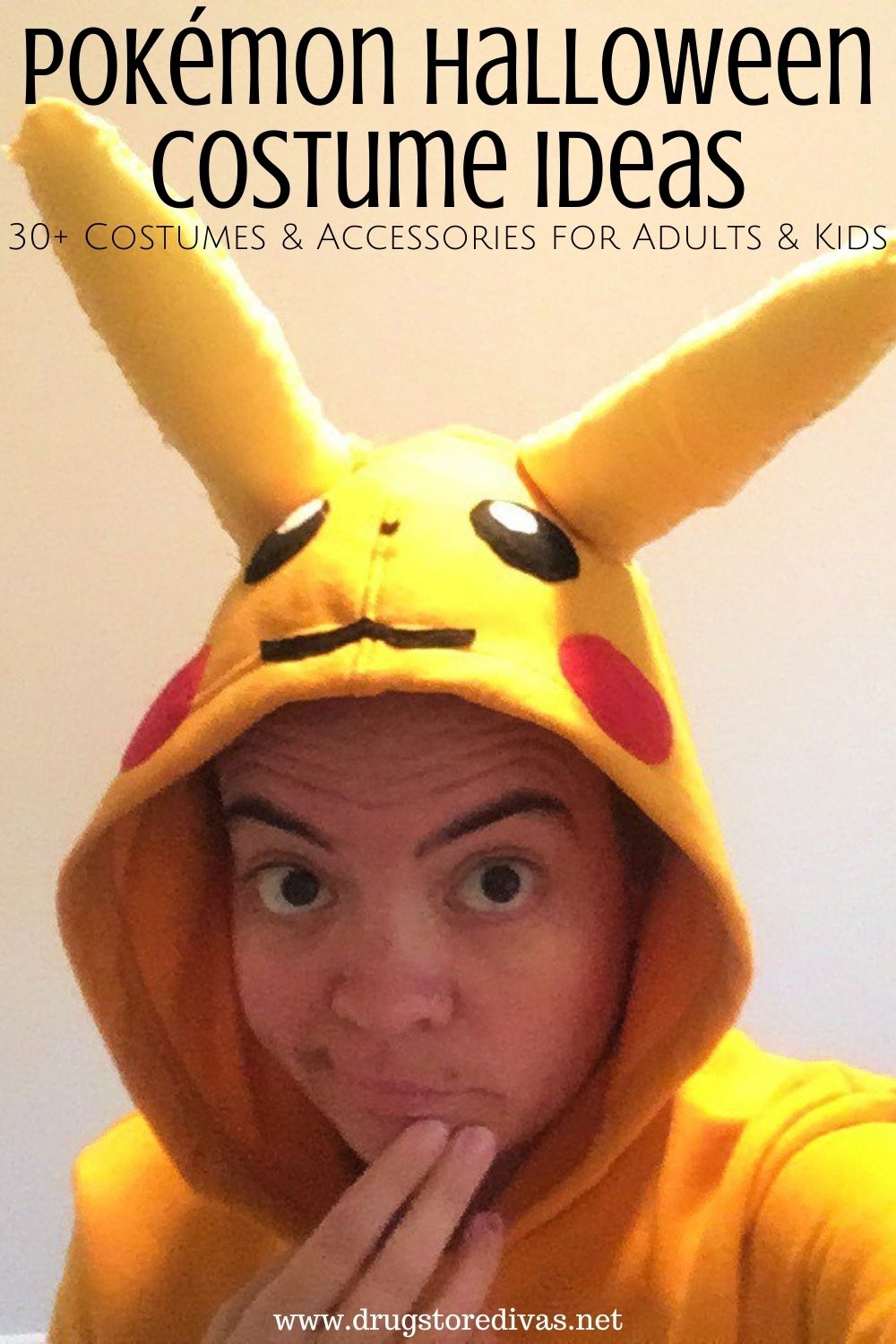In this image, we see a man wearing a yellow Pikachu onesie, embodying the iconic Pokémon character complete with a hoodie featuring Pikachu's large black eyes, big yellow ears, and distinctive red cheeks. His wide, surprised eyes, raised eyebrows, and thoughtful hand on his chin give him a curious, pondering expression. The background is a plain white wall, making the yellow costume stand out prominently. Text overlaid on the image reads "Pokemon Halloween Costume Ideas" at the top, with "30+ costumes and accessories for adults and kids" in smaller text beneath it. At the bottom of the image, there's a website link: www.drugstoredivas.net, indicating it's likely a promotional or marketing image for the site, potentially on platforms like Pinterest.